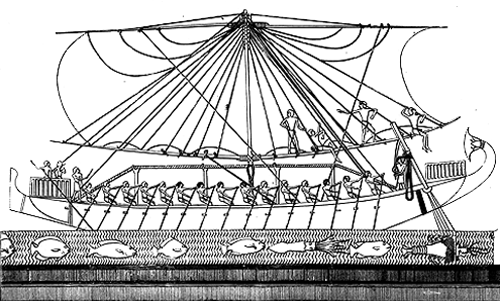This detailed black-and-white drawing depicts an old-school ship, likely powered both by paddling and wind. The ship's masts are adorned with rigging, and several individuals are seen sitting on elevated platforms working on the sails, ensuring they catch the wind properly. The main deck is crowded with approximately 10 to 15 rowers, possibly slaves, who are using long paddles that extend into the water to propel the vessel. A figure at the front appears to be giving orders to these rowers, while another figure in the back is seen with a long pole, potentially for navigating or pushing off from a dock. Complementing the maritime theme, the lower section of the drawing features an array of sea life, including fish and a lobster, adding an artistic and decorative element to the overall image.